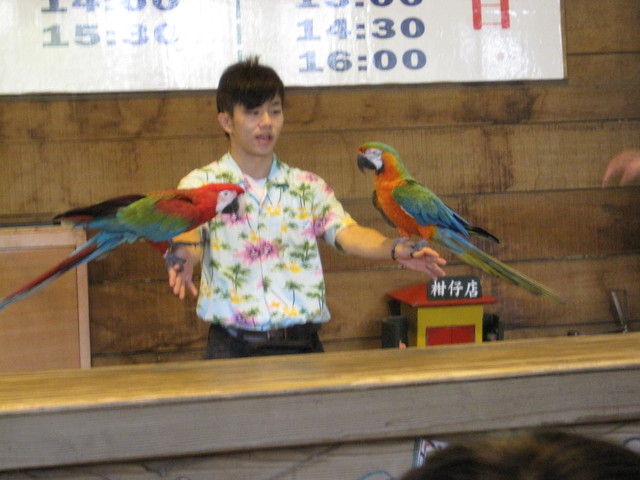This color photograph features an Asian man in his mid-twenties with short black hair, wearing a vibrant shirt adorned with green, purple, and yellow floral patterns on a white background. With his arms outstretched, the man is presenting two large and vividly colored macaws perched on his hands. The macaw on his right hand features a striking red head, green on the top of its head, and blue tail feathers, whereas the macaw on his left displays a yellowish-orange chest, with blue and green wings, and a similar colorful plumage. The man appears to be participating in a bird show or competition, as indicated by his engaged demeanor and slightly open mouth, suggesting he is speaking. In the background, there is a wooden wall, a white sign with blue numbers (including 1400, 1430, 1530, and 1600), and a small wooden box with Chinese or Japanese writing on it. In the foreground, there is a long walnut-colored table, and faintly visible at the bottom right is the crown of a spectator's head.